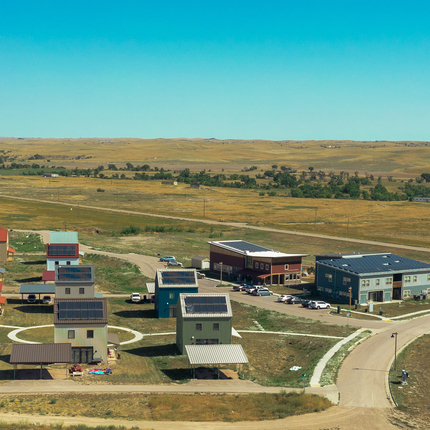This is a detailed vertical, rectangular photograph capturing a complex scene of various buildings, a road, and a landscape. The top third of the image features a turquoise sky that gradually fades to lighter shades toward the horizon. Below the sky, in the background, there's a desolate stretch of land characterized by patches of green and brown grass, with some telephone poles or lights dotted across it.

In the middle of the photograph, a variety of buildings and structures come into focus. Central to this scene is a large building with a distinctive light blue front, divided midway by a cyan color, and topped with a black roof. Adjacent to this building on the left is a line of parked cars, with a red building sporting a dual-colored roof—white on the right and black on the left—in the foreground. To the left of this red building stands a small barn, followed by two additional cars.

Each building in the foreground appears to have slanted roofs equipped with black solar panels arranged in two parallel rows. Notable among these structures is one with a maroon roof further back, and a carport with two parked cars beneath a dark blue roof. Another carport nearby is silver, sheltering a white car. The buildings exhibit a variety of colors: beige with a dark blue roof, dark blue with a silver roof, and olive green with both brown and silver carports.

The road infrastructure includes a large dirt road on the right side which transitions to a paved road. This road curves around, forming a circular pattern that connects to a sidewalk running alongside the main thoroughfare. At the terminus of the sidewalk, another road intersects, passing in front of two additional buildings with olive green fronts and brown roofs.

In the foreground extends an expansive, yellow-green field with a faint gray undertone, bordered by a distant line of green trees. The scene is captured in natural daylight, enhancing the visibility of the details, from the precise colors of the roofs to the positioning of the solar panels and parked cars.